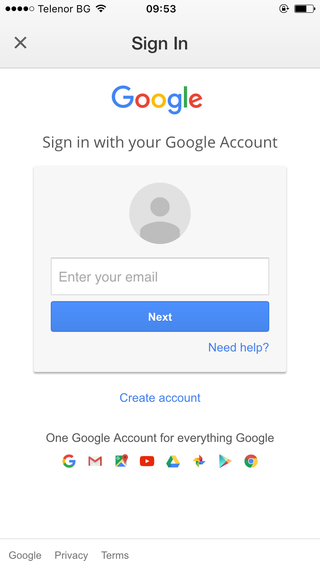This is a screen capture taken from a mobile device displaying the Google sign-in page. At the top of the screen, there's a rectangular status bar showing the mobile network name "Telenor BG" on the left, with the Wi-Fi signal icon next to it. The time, "9:53," is centered, and a battery icon indicating half charge is on the right. 

Below the status bar, the page header includes the text "Sign in" in black, with an "X" on the left to close the page.

On the main body of the page, against a white background, the vibrant multicolored Google logo is prominently displayed. Beneath it, in grey text, is the instruction: "Sign in with your Google account." Following this, a grey square box features a centered light grey circle with a dark grey stylized image of a person, indicating that no account is currently selected.

Below the box, a white text field labeled "Enter your email" in light grey invites users to input their credentials. A blue rectangular button with "Next" written in white text is located beneath the text field. "Need help?" is written in blue just below the "Next" button.

Moving further down, the text "Create account" appears in blue, offering users the option to establish a new Google account. Directly below, still on a white background, the black text states, "One Google account for everything Google," accompanied by icons of various Google products representing the breadth of services that can be accessed with a single account.